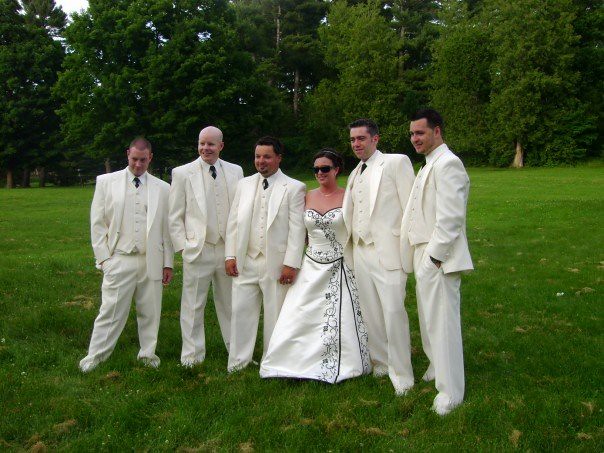In a lush, verdant lawn framed by mature hardwood trees with sunlight filtering through their canopies, stands a wedding party. The expansive green grassy field, dotted with a few fallen leaves, creates a picturesque backdrop for the scene. Six individuals are lined up, gazing towards the left side of the frame. Five men, dressed in immaculate white suits—comprising white jackets, vests, shirts, pants, and shoes—complement their outfits with black neckties tucked into their vests. The first man on the left sports closely cropped hair with a widow's peak, followed by a tall, light-haired or possibly bald man. The likely groom stands third, discernible by his stature, slightly darker skin tone, dark hair, mustache, and beard; he wears a wedding ring. Next to him is the bride, adorned in an elegant strapless white gown with black piping and embroidered floral details, her hair pulled back and accessorized with black sunglasses. Completing the group are two more groomsmen, both tall with dark hair and squared-off haircuts. Against the serene and natural setting, their coordinated attire and subtle poses encapsulate the classic elegance of an outdoor wedding.